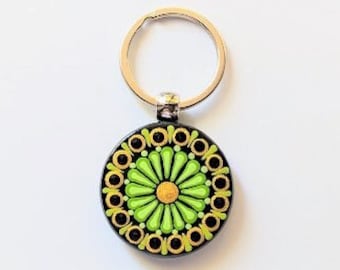The image depicts a circular keychain featuring a beautifully intricate design. At the center of the keychain is a vibrant flower with a yellow center surrounded by approximately 16 slender lime green petals. Encompassing the flower is a delicate blue outline adorned with circular petal patterns, enhancing the central flower's striking appearance. The outer edge of the keychain is decorated with yellow and black circular patterns, interspersed with tiny white beads giving it an elegant finish. The keychain is positioned atop a white surface, which accentuates the vivid colors and intricate details of this pretty trinket. At the top, a gold hoop allows it to be attached to a key ring, necklace, bracelet, or any item requiring a decorative pendant.